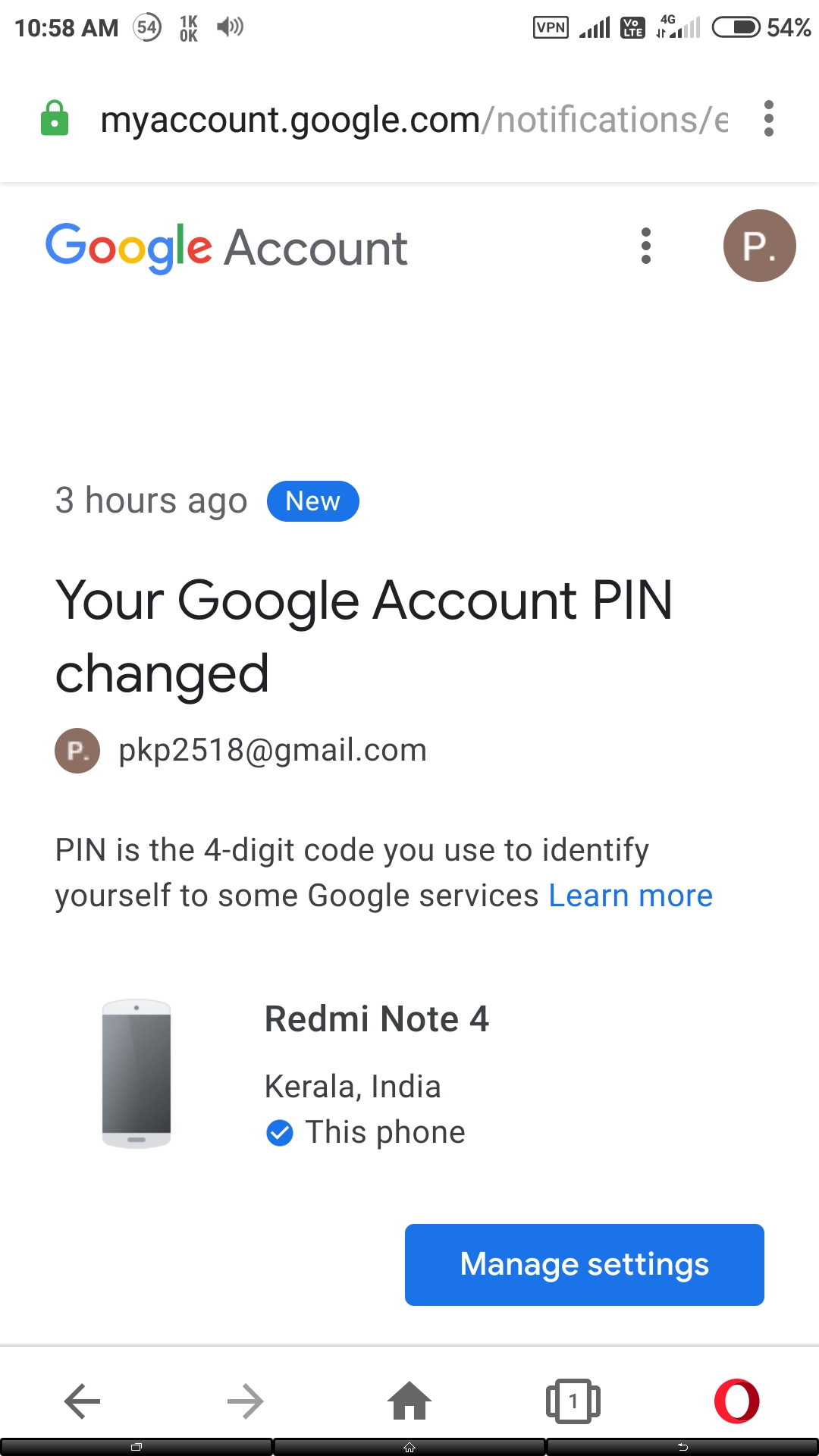This screenshot, taken from a smartphone, has a white background and displays various status icons and a notification message. In the top left corner, the time reads "10:58 a.m." adjacent to a small circle displaying "54." Following that, there is a "1K" over "0K" label, a volume icon, and, on the far right, a square indicating "VPN" status. The signal strength is shown through five fully filled black bars next to the "4G" symbol, with a battery indicator showing 54% remaining.

Below the status bar is a green padlock icon next to a notification text reading "myaccount.google.com notifications." The next line includes "Google account" followed by three vertical dots and a brown circle with the letter "P."

Further down, there is a blank white space, followed by text stating "three hours ago" in the vicinity of a blue oval shape labeled "new." The notification specifies that "Your Google account PIN changed" with an accompanying email address "pk2518@gmail.com." This email is denoted by a brown circle with a "P" inside it. The notification explains that a PIN is a four-digit code used to identify oneself to some Google services, with a "Learn more" link in blue text.

Beneath this explanatory text, there is an image of a phone displaying "Redmi Note 4, Kerala, India" with a checkmark labeled "this phone." At the bottom of the screenshot, a blue button reads "Manage settings."